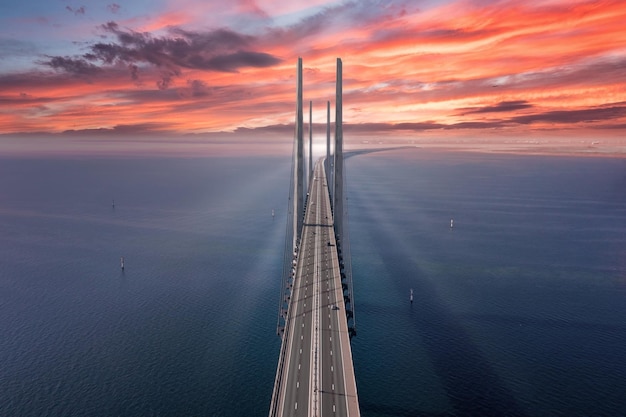This photograph captures a breathtaking scene of an expansive bridge stretching out into the horizon over calm, clear blue waters. The bridge, featuring two lanes of traffic in each direction and accented by very tall posts, dominates the composition, extending straight down the middle of the image before curving slightly to the right at the horizon. The setting, either at sunrise or sunset, bathes the partly cloudy sky in stunning pink, purple, orange, and red hues, with a touch of blue peeking through the clouds. A bright, white light source near the center casts radiant rays over the bridge and water, enhancing the tranquil ambiance. There are no signs of land or boats in the picture, just a few cars driving on the bridge and a couple of pillars jutting out of the still water, completing this serene and picturesque scene.